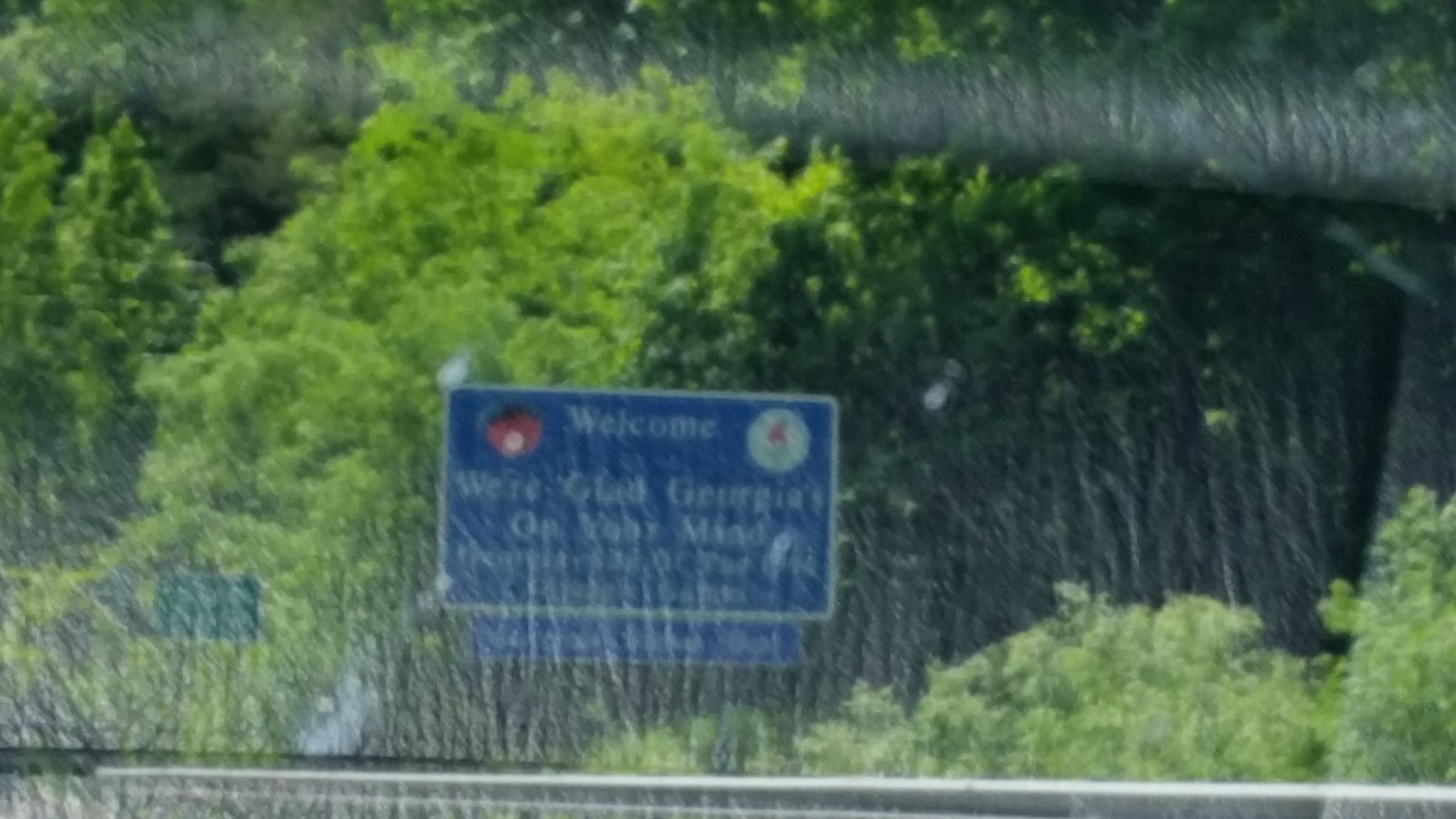In this image of the outdoors, presented in a rectangular format, the overall quality is notably low. The picture appears blurry and fuzzy, characterized by its low resolution, making it difficult to discern finer details. Despite the poor quality, a prominent blue rectangular sign can be seen in the middle of the image. This sign features white text, with "Welcome" being the only legible word due to the blurriness obscuring the rest. Below this primary sign, there is a smaller rectangular sign, also displaying white text, though the content is equally unreadable. The combination of these elements hints at an entry or informational point, even if the specifics remain unclear.